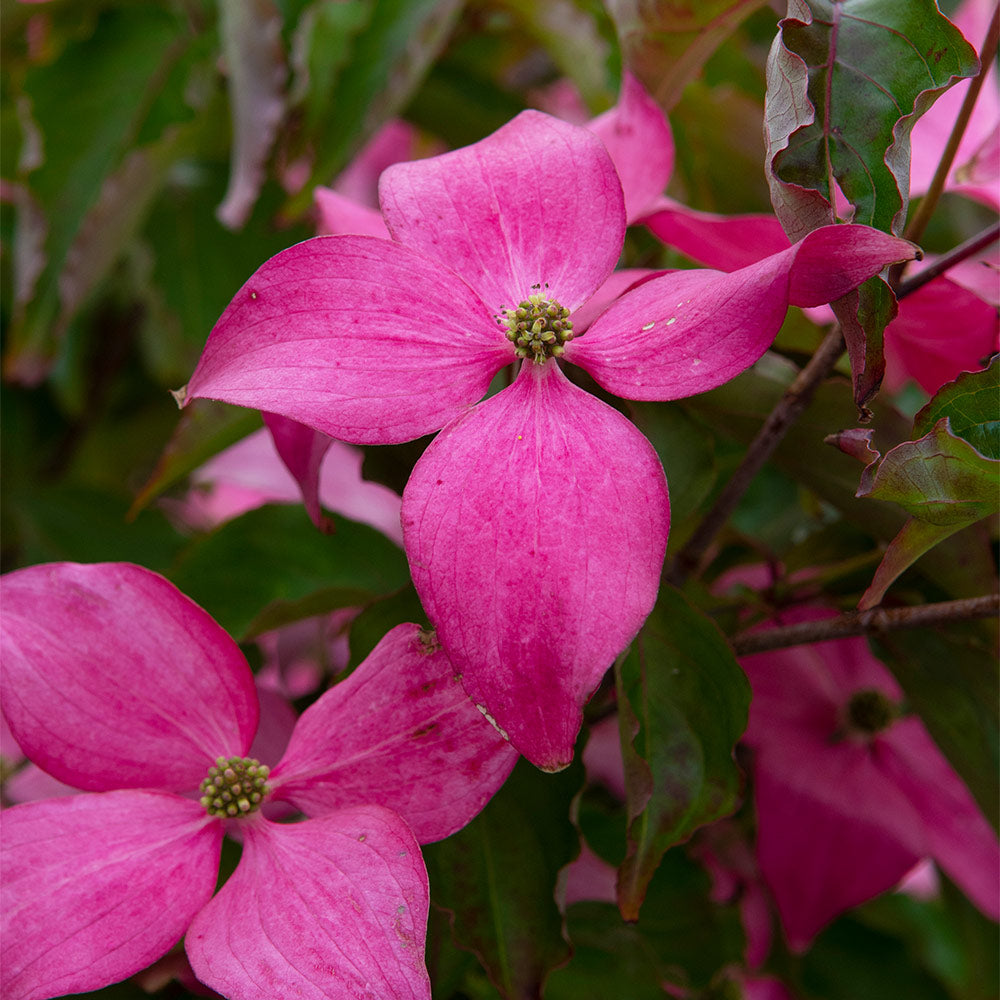This image is a detailed close-up of two identical flowers in full bloom. Each flower, with its four broad petals, displays a stunning light pink hue accented by darker pink veins. At the center of each bloom, clusters of bright yellow and green stamens form intricate, eye-catching patterns. The photograph’s focus is sharply centered on these two flowers, making their delicate structure the main highlight, while the background remains artistically blurred. The backdrop contains green leaves and additional flowers, subtly indicated by blurry corners and faint outlines, with a few more pink flowers hinted at beneath the primary ones. The composition suggests a refined nature photography style that beautifully draws attention to the vibrant details and natural beauty of the flowers.